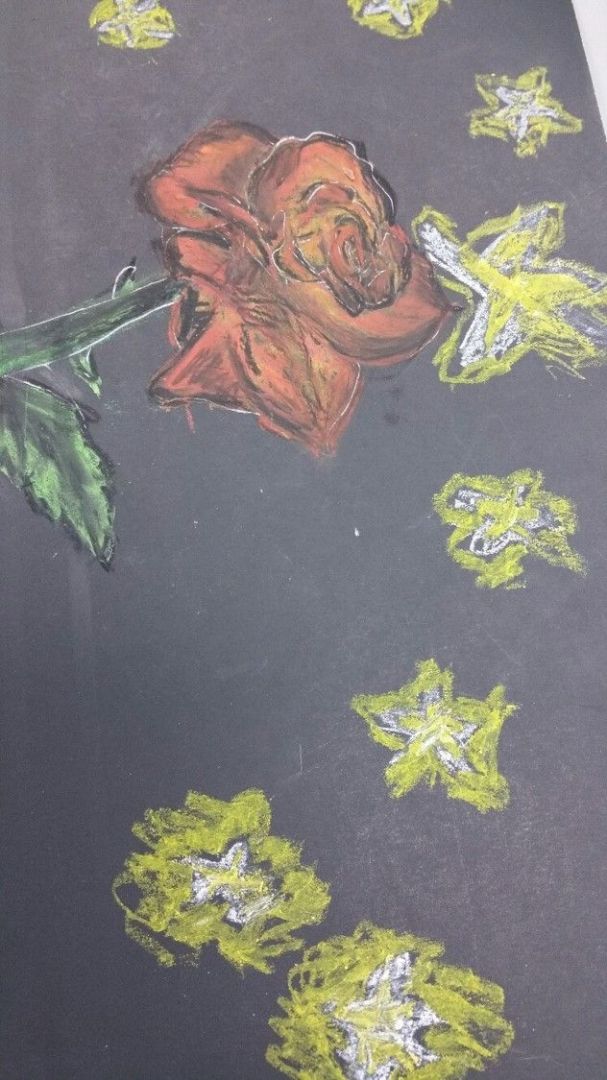A beautifully detailed chalk drawing adorns a black chalkboard background. At the center, a realistic rose rendered in vibrant hues of red, yellow, and orange captures the eye. The flower features sketchy yet precise white and black outlines that accentuate its intricate petals. This striking rose extends horizontally from the left side of the image, supported by a green and black colored stem adorned with two sharp thorns and a single verdant leaf. Surrounding the rose, a constellation of yellow and white stars twinkle softly, adding a touch of whimsy and enchantment to the composition.